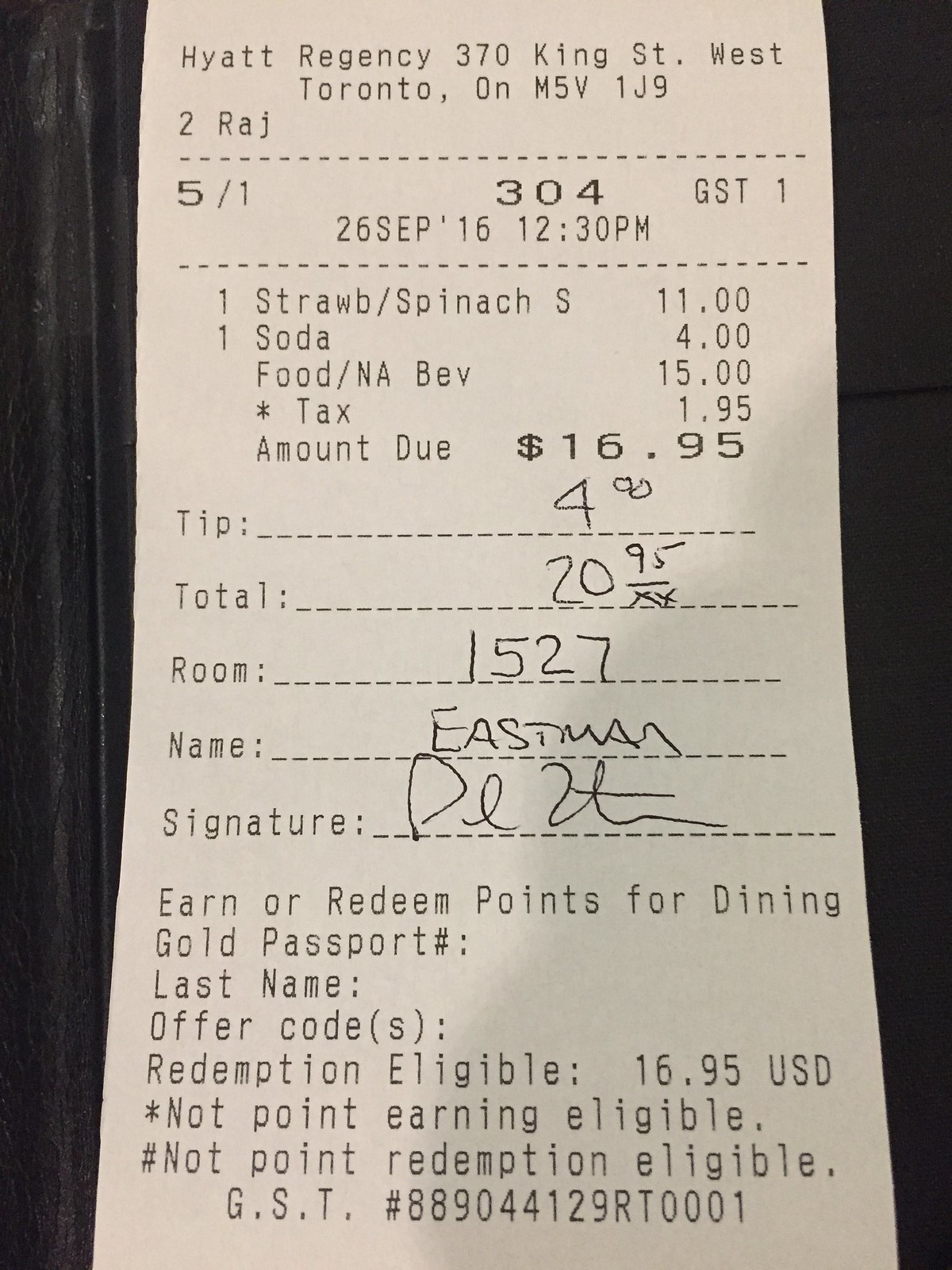This black-and-white photograph captures a receipt from the Hyatt Regency Hotel located at 370 King Street, West Toronto, ON. The receipt, detailed with plain black computerized text, documents a lunch purchase made on September 26, 2016, at 12:30 PM. Items listed include a strawberry spinach salad for $11 and a soda for $4, totaling $15. With an added tax of $1.95, the total amount due came to $16.95. The receipt shows a handwritten tip of $4, bringing the final billed amount to $20.95. The charge was billed to room 1527, registered under the last name Eastman, accompanied by an unreadable signature. The bottom of the receipt includes details about earning or redeeming points for dining with a Gold Passport, although it mentions that this particular transaction is not eligible for point earning or redemption. Supplemental details include the GST number 889044129RT0001 and a special note for redemptions eligibility of $16.95 in USD. The receipt is placed against a black background, with a half-inch margin on the left and varying from a one-inch to half-inch margin on the right.